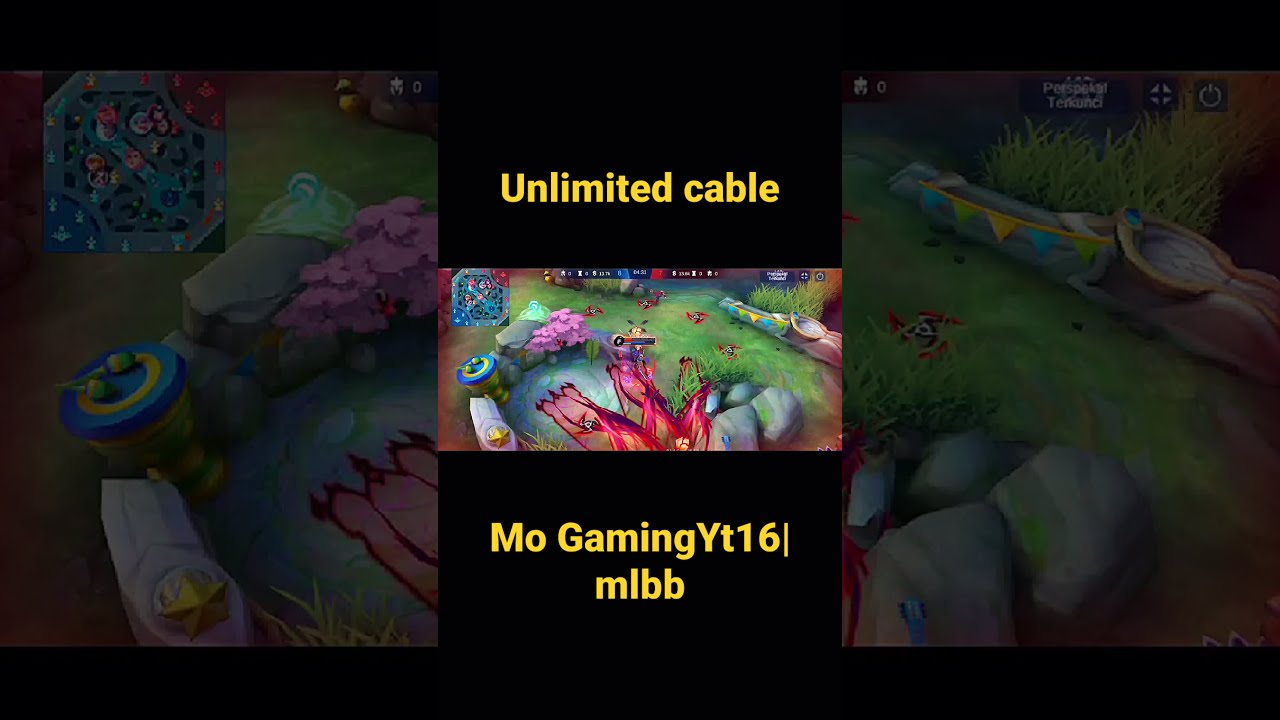This horizontally aligned rectangular image is a clip from a video game that appears to serve as an advertisement for a YouTube channel. Central to the image is a vertical rectangle flanked by thick solid black borders at the top and bottom. The top border features yellow text that reads "Unlimited Cable" while the bottom border displays "MoGaming YT16 MLBB" in similar yellow print. Within these borders, the main in-color screenshot reveals a game scene dominated by a green and blue field with scattered rocks, some water, and vibrant flowers. The image includes a detailed visual element showing the back end of a nine-tailed fox and numerous targeted points scattered across the grassy area. Flanking this central image, the left and right sections contain blurry close-ups of the game's elements, enhancing the visual information. On the left, there's a focus on the flowers and water, while on the right, there’s an emphasis on the grass and rocks. Overall, this snapshot provides an engaging and colorful depiction of the game environment, potentially promoting the MoGaming channel’s content.